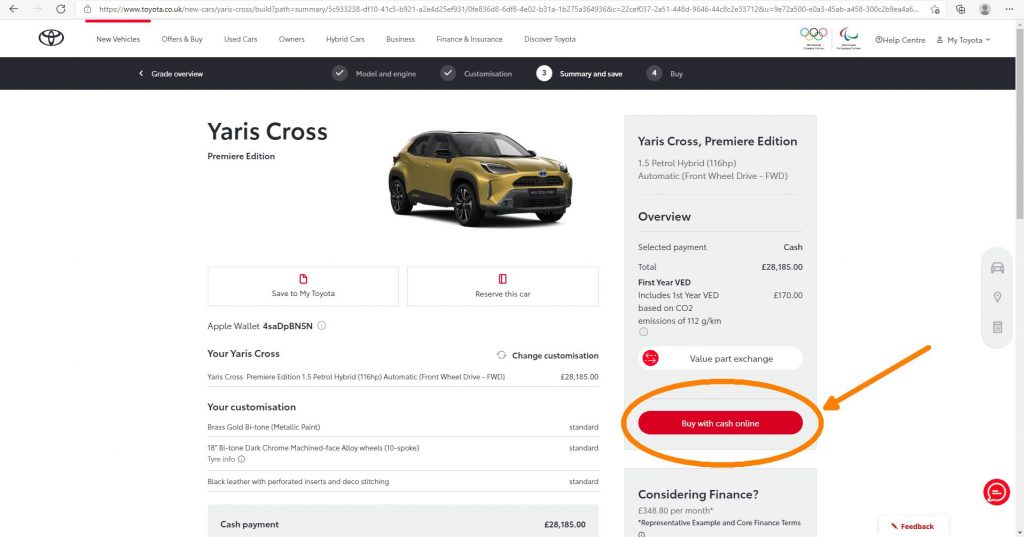The top section of the website features a predominantly white background. On the left side, there is a black arrow pointing left, a gray arrow pointing right, and a refresh icon that appears circular. The web browser bar is also white, displaying “https://www.toyota.co.uk” in gray text, underlined in red for reasons unspecified. To the left, the Toyota logo is displayed in black, accompanied by black text listing various sections: "New Vehicles," "Offers," "Buy Used Cars," "Owners," "Hybrid Cars," "Business," "Finance and Insurance," and "Discover Toyota." Additionally, options for "Help Center" and "My Toyota" are also present.

Continuing towards the top within a black border, white text states the current navigation steps: "Overview," "Model and Engine," "Summary and Save," with "Save" highlighted to indicate the current step, and "Buy" noted as the final step. Below this, the main content showcases a Yaris Cross Premier Edition car in an olive color. Beneath the vehicle's image, options to "Save to My Toyota" and "Reserve This Car" are provided, alongside an Apple Wallet link for the car identified by the code SADPBN5N. To the right, a red oval button with white text offers the option to "Buy with Cash Online," accentuated by an orange oval and pointing arrow for emphasis.